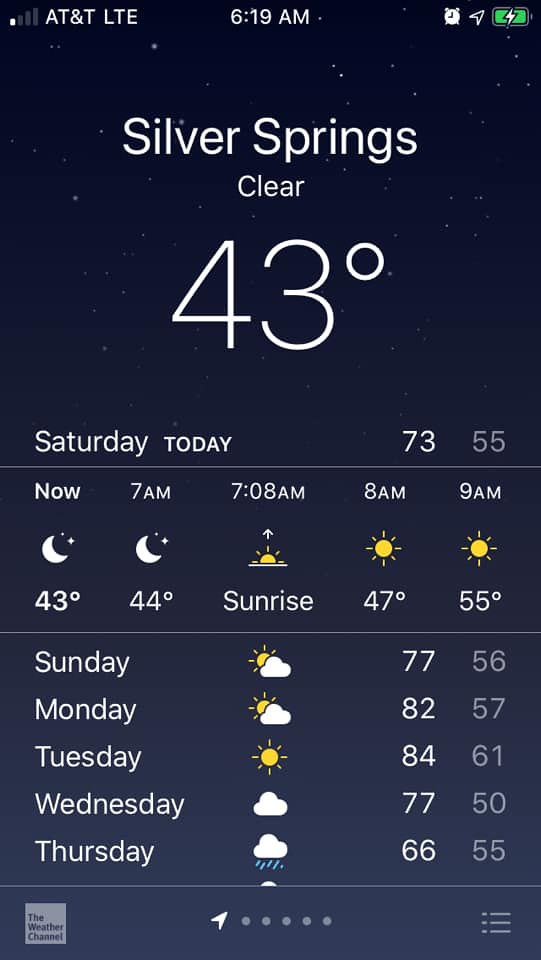This image captures a detailed weather forecast displayed on a smartphone screen. The top indicates the carrier AT&T LTE on the left, the time 6:19 AM in the center, and icons for an alarm clock, an arrow, and a green battery symbol in the upper right, suggesting the phone is charging. The background of the app is dark blue. Prominently featured is the location 'Silver Springs,' where it's currently clear and 43 degrees. Below this, 'Saturday, today' indicates a high of 73 degrees and a low of 55 degrees. A detailed hourly forecast follows, with a half moon icon and 43 degrees for 'now,' 44 degrees at 7 AM with a moon and an arrow pointing upwards for 'sunrise' at 7:08 AM, 47 degrees at 8 AM depicted with a full sun, and 55 degrees at 9 AM also with a full sun. At the bottom of the screen, a weekly forecast is displayed. Sunday shows a partly cloudy icon with temperatures 77/56, Monday the same with temperatures 82/57, Tuesday a sun with 84/61, Wednesday a cloud with 77/50, and Thursday a rain cloud with 66/55. The bottom left corner features a square icon for 'The Weather Channel,' the center bottom displays a white arrow pointing up and five grey dots, and on the far right, there are three vertical lines stacked on top of each other.